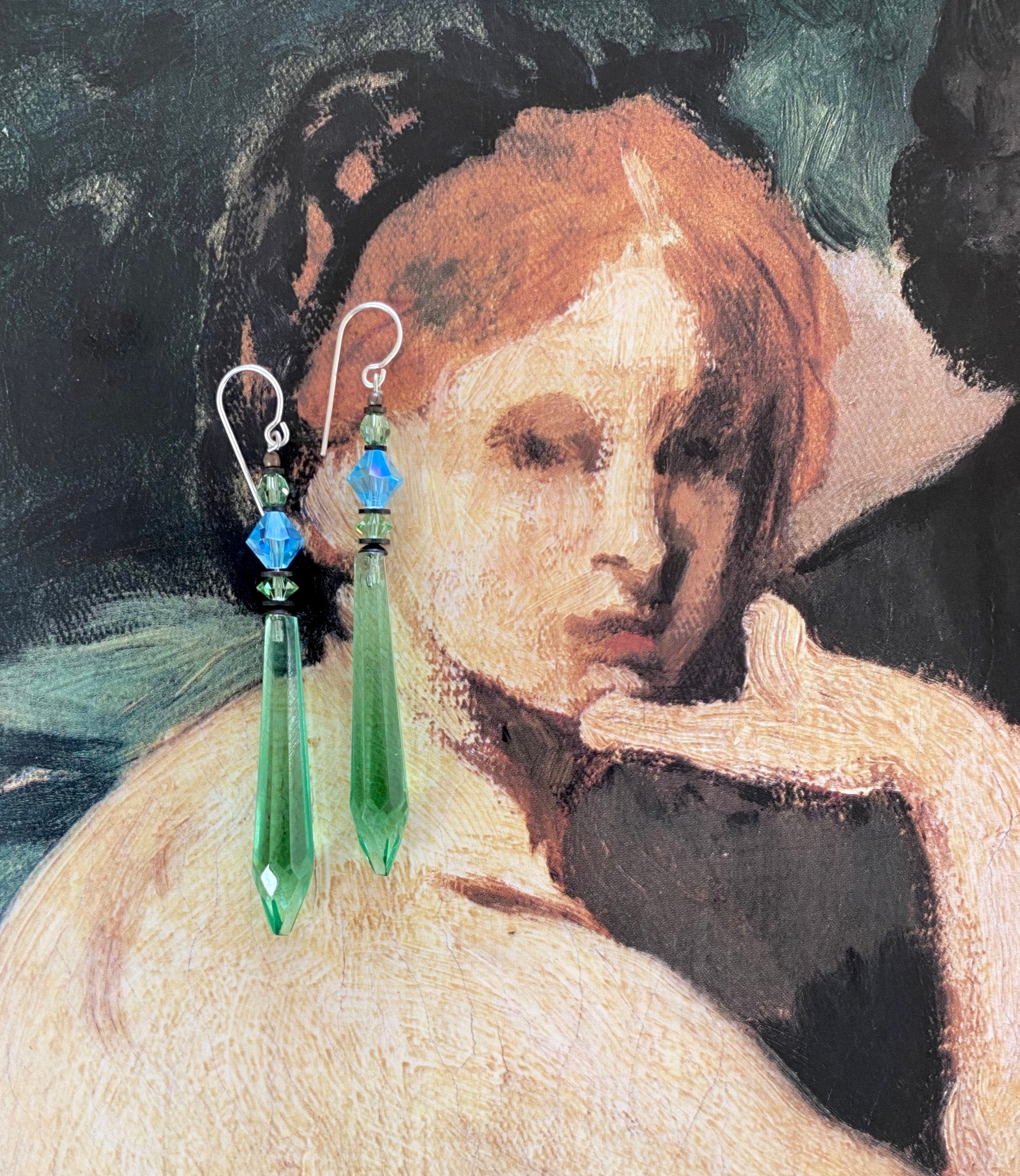The image features an impressionistic watercolor painting of a red-haired woman with her hair pulled up, adorned with a black bonnet. The painting, showcasing the woman's bare back and subtle facial features, presents her body facing to the right while she looks over her shoulder towards the camera with her hand resting by her chin. Superimposed over the painting, and serving as the focal point of the image, are a pair of long, dangly earrings made of alternating green and blue crystal beads. The earrings, positioned near the woman's depicted ear, are detailed with elongated green teardrops, blue stones, and additional green stones, suggesting they might be the subject of an advertisement.